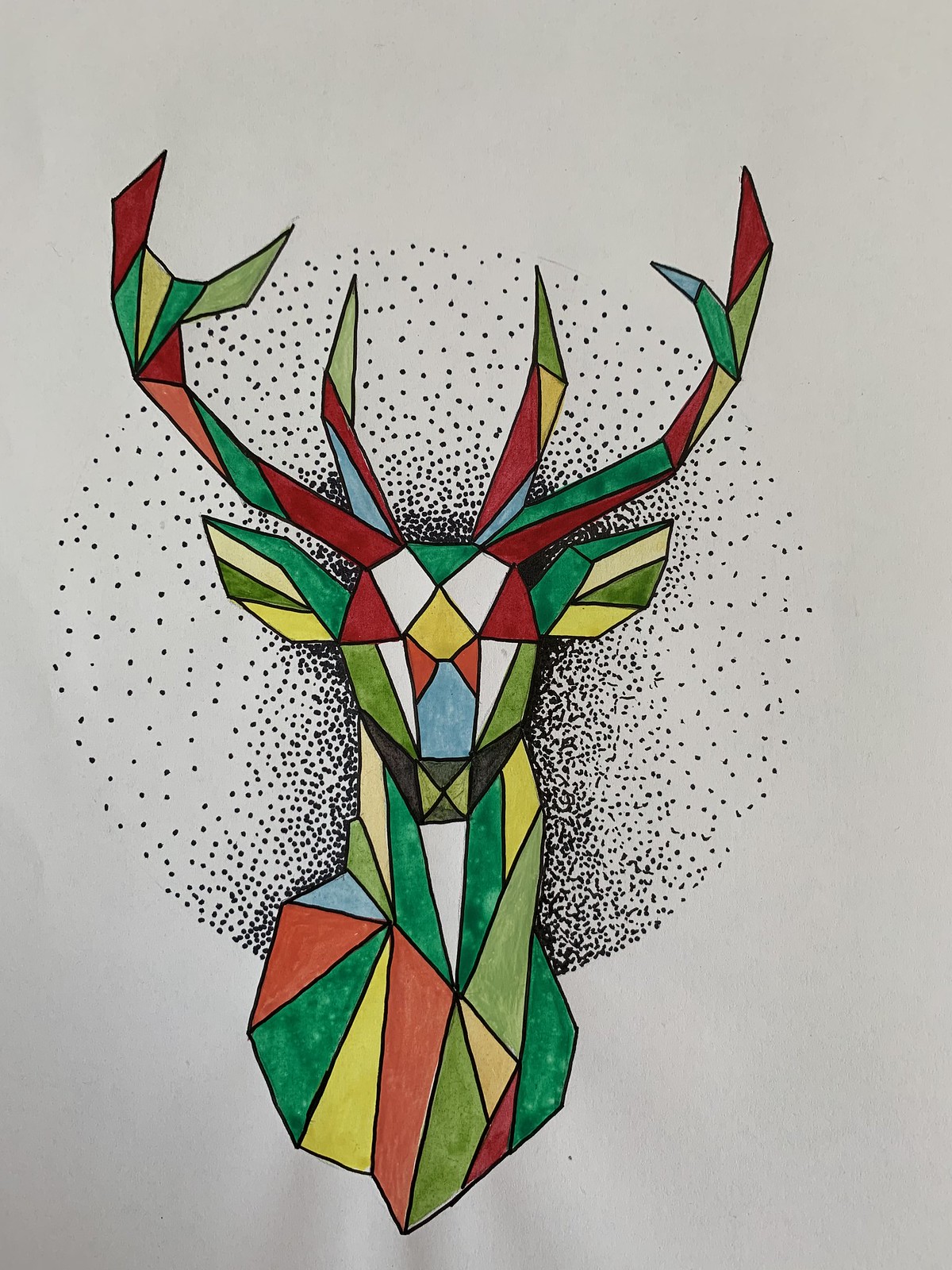The image features a striking depiction of a deer's head and neck, crafted entirely from a mosaic of angular geometric shapes, reminiscent of stained glass. The deer is adorned with a vibrant palette that includes light green, dark green, yellow, orange, magenta, red, black, blue, and various shades of tan and beige. Its antlers, distinct with six points, are primarily colored in red, while other geometric sections create a patchwork effect across the face, neck, and upper torso. Notably, the deer lacks eyes, its face instead composed of evenly divided hexagonal shapes. Surrounding the deer, a circular pattern of black dots originates from its antlers and extends to its shoulders. The density of these dots increases closer to the deer's outline, creating a gradation effect against the stark white background. The overall artistic piece combines elements of sturdy geometric design with a dynamic, colorful expression.